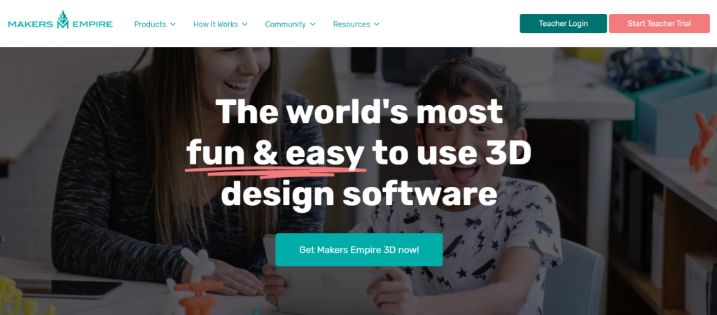In this image, the top section features a white header containing the Makers Empire logo. The logo comprises the words “Makers Empire” flanking a blue ‘M’, topped with a small diamond shape. Located beneath this logo are four dropdown labels: "Products," "How it Works," "Community," and "Resources," each with a downward arrow indicating additional options. On the right side of the header, two buttons are prominently displayed: one green button labeled "Teacher Login" and another pink button labeled "Start Teacher Trial."

Below the header, a large, central image showcases an engaged teacher sitting at a table with a young student. The teacher is holding some papers and appears genuinely happy as she interacts with the child. Both are engrossed in an educational activity. The caption overlaid on this image reads, “The world’s most fun and easy,” with the words "fun and easy" underlined multiple times in red for emphasis. Below this statement, a bold blue button invites the viewer to "Get Makers Empire 3D Now."